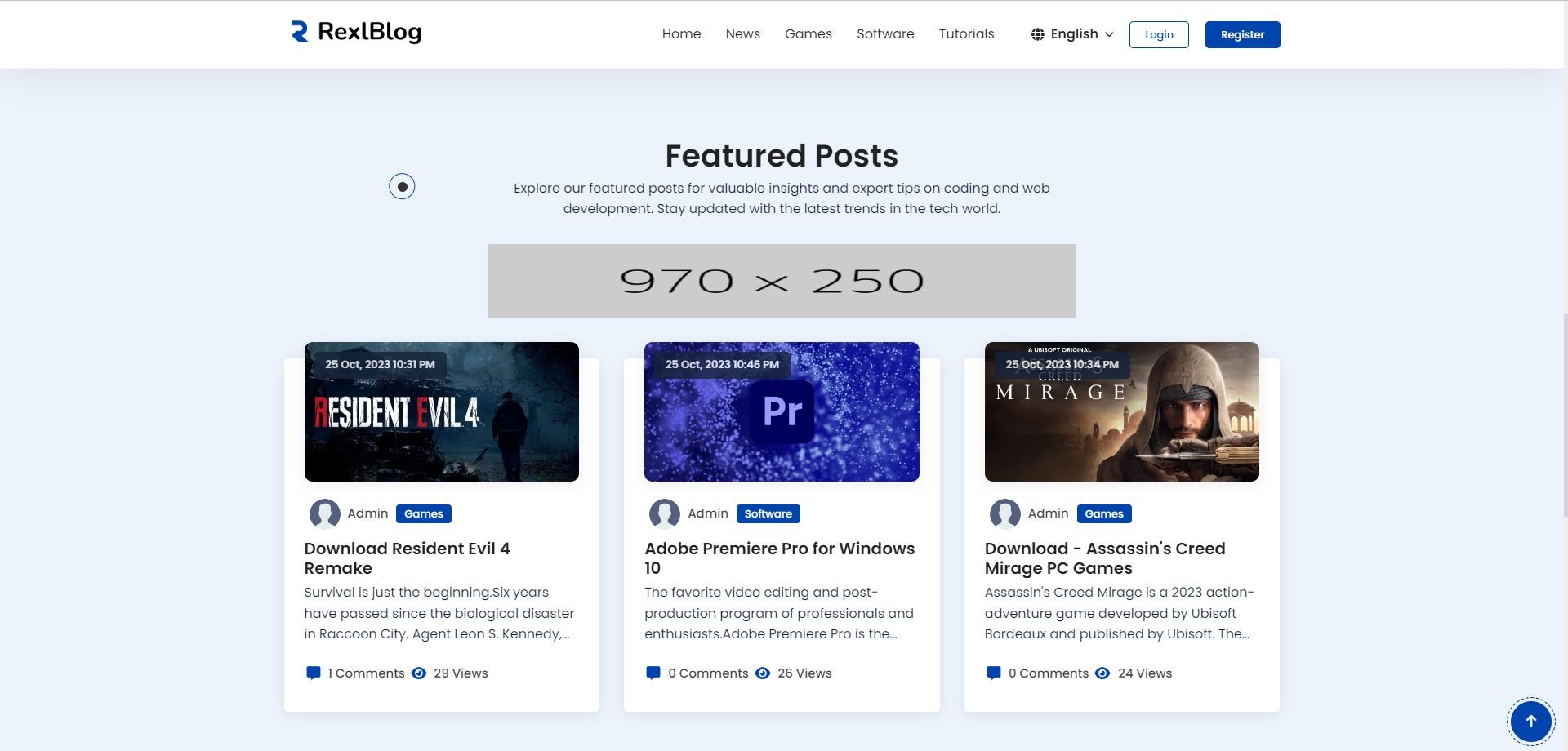The image is a horizontally rectangular screenshot of a website. The top section features a white horizontal banner with the Rexel blog logo on the left. As we move to the right, options for 'Home,' 'News,' 'Games,' 'Software,' and 'Tutorials' are listed, followed by a drop-down menu for language selection, currently set to English, and buttons for 'Login' and 'Register.' The background of the remaining frame is a pale light blue.

Centered in bold text, it reads "Featured Posts," accompanied by a subheading that states, "Explore our Featured Posts for valuable insights and expert tips on coding and web development. Stay updated with the latest trends in the tech world."

Beneath this, a gray horizontal rectangular banner displays the dimensions "970 by 250." Below this banner, there are three vertically rectangular windows aligned side by side, each containing an image at the top. The listings beneath these images are: "Download Resident Evil 4 Remake," "Adobe Premiere Pro for Windows 10," and "Download Assassin's Creed Mirage PC Games."